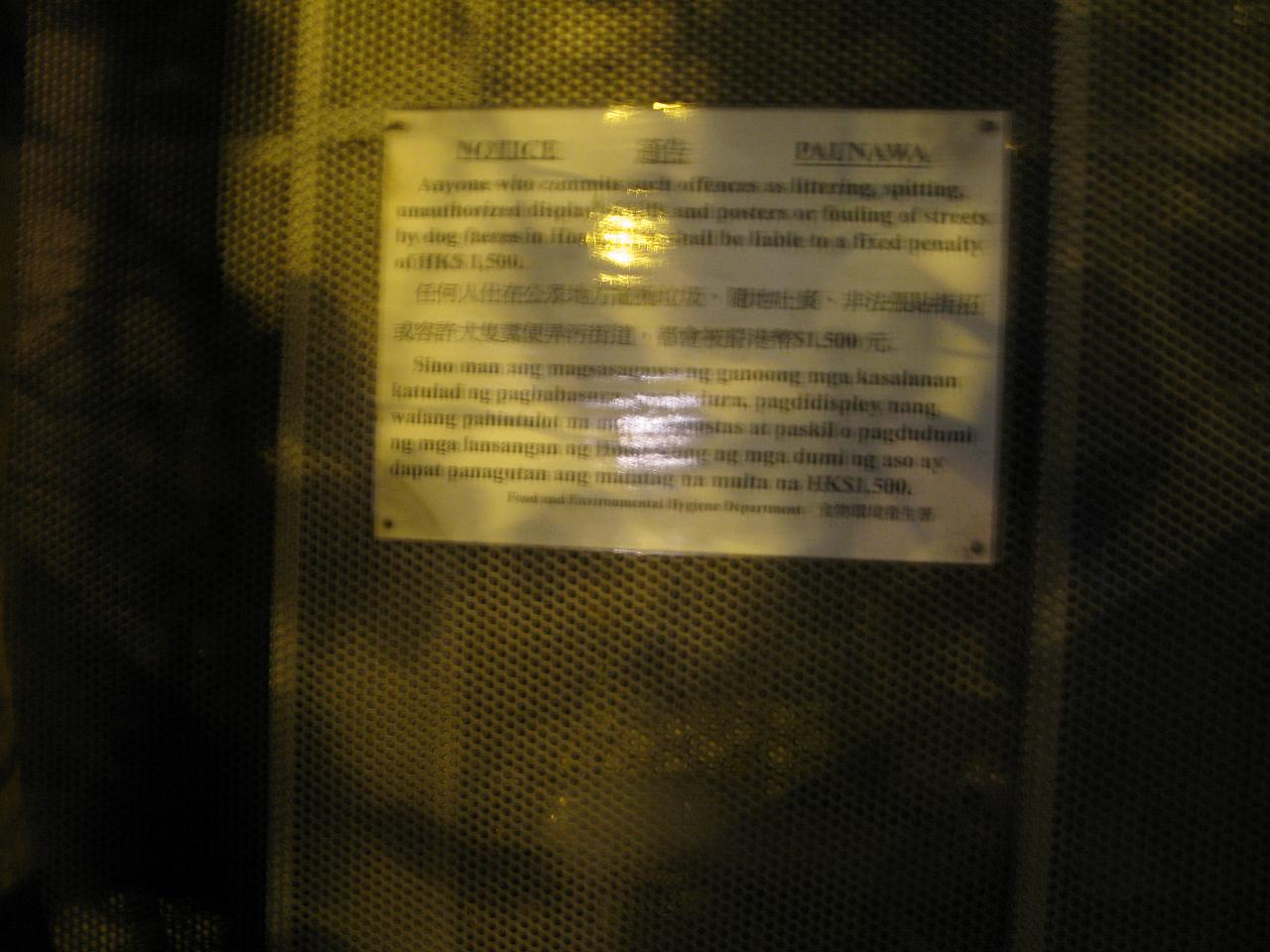In this nighttime outdoor image, a metallic mesh gate is visible, adorned with vertical lines and small perforated holes. Affixed to the center of the gate is a white sign secured at each corner with tacks or rivets, covered by a reflective plastic film. Despite parts being obscured by light reflection and blurriness, the sign prominently displays the word "Notice" underlined in black. The text, partially in English, warns against various offenses including littering, spitting, unauthorized display, and the fouling of streets by dog feces. It states that violators will be liable to a fixed penalty of HKS 1,500. Additionally, the sign features Chinese characters and the word "Paonawa" at the top, suggesting multiple languages, potentially indicating a location in China, Hong Kong, or Taiwan. The mesh gate prevents any clear view of what lies behind it.